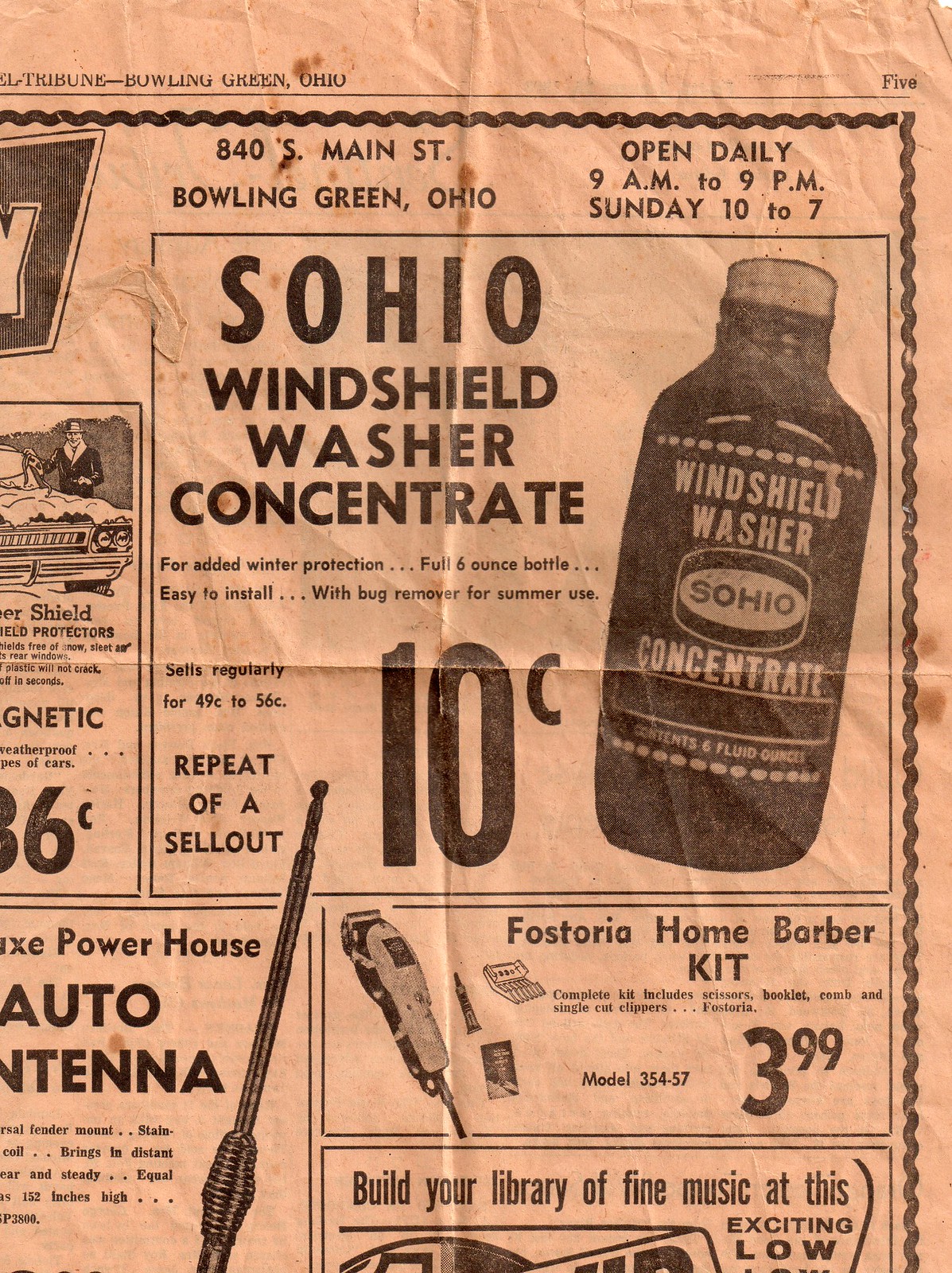The image depicts a highly creased and yellowed page from an old edition of the Tribune newspaper, specifically from Bowling Green, Ohio. The page, marked as Page 5, predominantly features various advertisements. Prominently positioned in the top right corner is an ad for Sohio Windshield Washer Concentrate, marketed for added winter protection and summer bug removal. The product is a full six-ounce bottle, regularly priced between 49 and 56 cents, but currently offered at a deeply discounted price of 10 cents. The ad includes a clear illustration of the bottle, highlighting its contents of six fluid ounces. Below this, there's an advertisement for the Fostoria Home Barber Kit, which includes scissors, a booklet, a comb, and single-cut clippers, priced at $3.99 and referred to as model 354-57. Another partially visible ad mentions building a library of fine music at an excitingly low price, but the details are cut off. On the left-hand side, there's an ad for a Powerhouse Auto Antenna, along with another for windshield protectors. The entire page is characterized by its aged appearance, with noticeable reddish-orange-yellowing and brown stains, adding to the vintage charm of the newspaper, likely dating back to the 1950s or earlier.